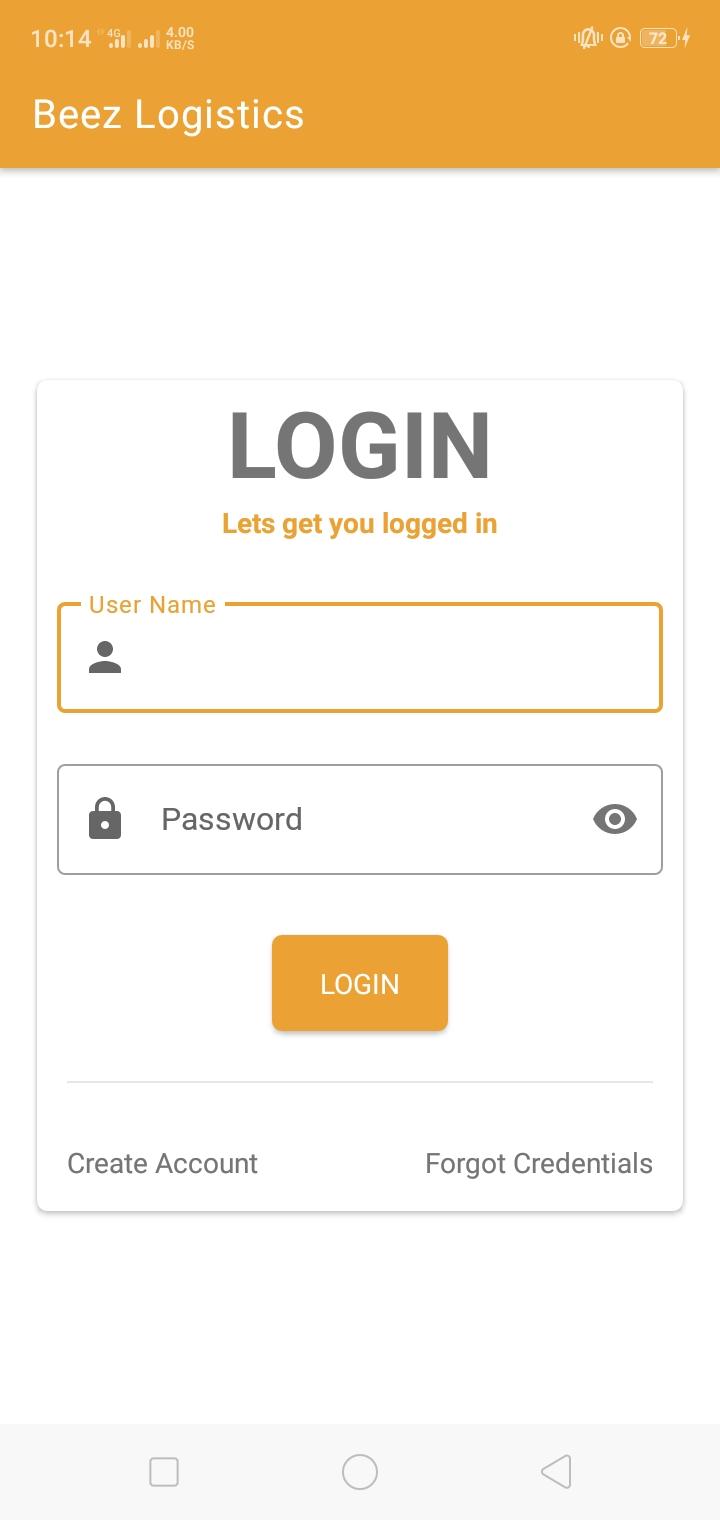The image depicts a phone screen displaying the login page of an app named "Bees Logistics." The device is connected to a 4G network, as indicated by the signal icon in the top left corner, and has 1014 gigabytes of storage available. The phone is set to vibration mode, with no notifications currently visible, and the screen rotation feature is enabled. The battery level is at 72%.

The login page features an orange background with white text and logistical information. Centred on the screen, the title "Login" is displayed in bold, grey text. Just below, an encouraging message reads, "Let's get you logged in," in orange lettering.

The username input field is outlined in orange and accompanied by an icon of a person, suggesting where users should input their username. Below the username field is the password input box, which remains grey until interacted with. This box includes an icon of a lock and the word "Password" in grey lettering, along with an eye icon to toggle password visibility.

An orange button labeled "Log In" in white text is located at the bottom of the fields. Below this button, users have the options to "Create account," written in grey text, and "Forgot credentials," also in grey, positioned to the right of the "Create account" text. The entire interface is designed to facilitate user access to the Bees Logistics app.